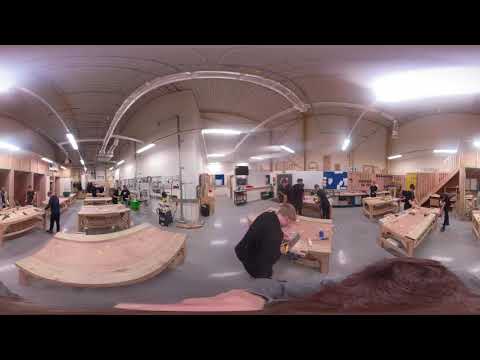The image depicts a vast construction warehouse or woodworking shop bustling with activity. The setting features a gray concrete floor and numerous wooden workbenches scattered throughout the space, each bolted together and hosting various tools and materials. At the center of the image, there is a woman with short blonde hair, dressed in all black, who appears to be sewing or working with a plank on a table that has blue tape on it. To her left, a team of three dressed in black collaborates at another bench, possibly drawing or planning. Nearby, another individual works alone at a table oriented towards the bottom right of the scene. In front, two more individuals are cutting materials at the edge of their workstations. Further to the left, another trio is engrossed in their tasks, while two men stand beside a green box, perhaps preparing to start a new project. The ceiling lights cast reflections onto the ominous gray floor, and the layout includes some stairs, computers, and doors in the background. The photograph, captured with a fisheye lens, exaggerates the scale of the warehouse, adding a slight curvature to the scene. The overall atmosphere suggests a productive day in this functional yet unassuming workspace.